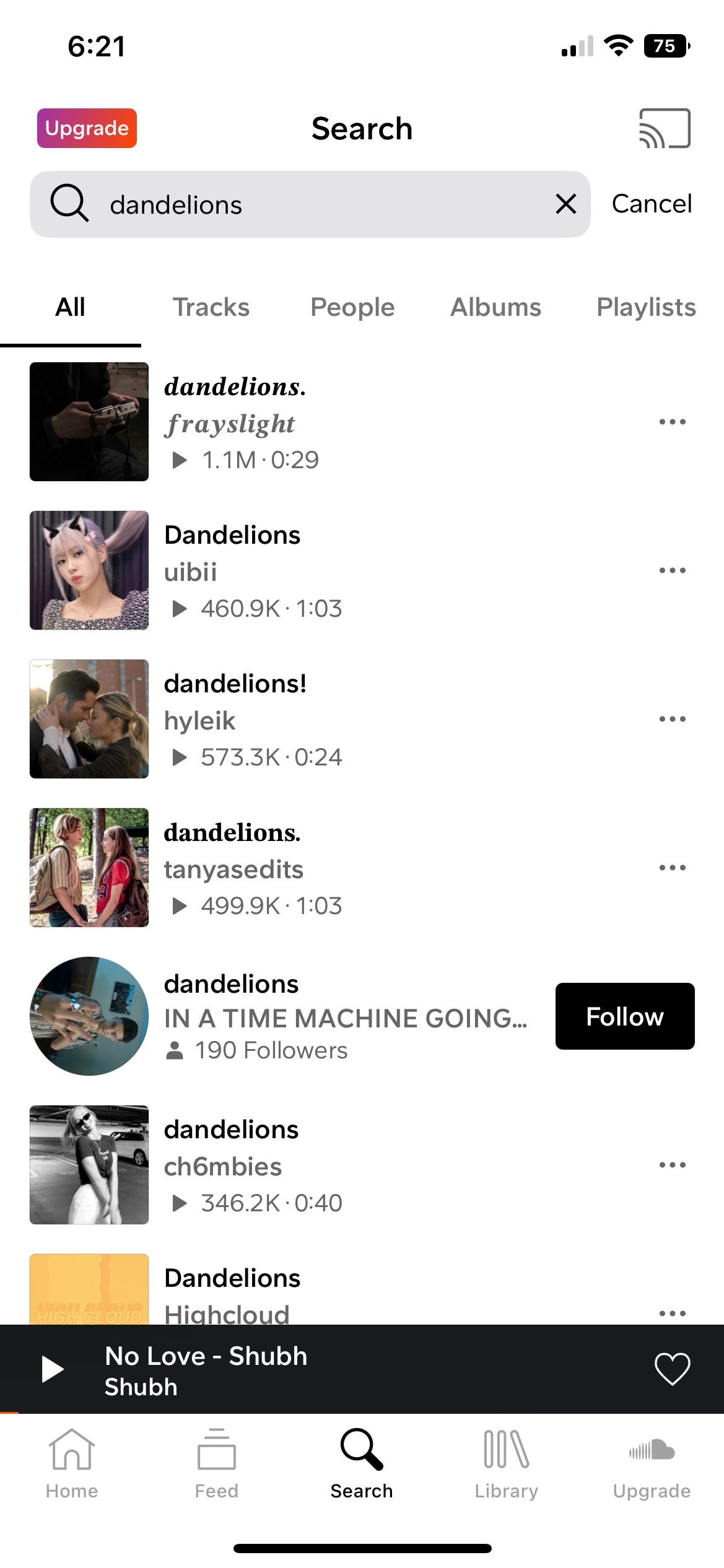The image depicts the search page of a music streaming application on a mobile device, likely a cell phone, in portrait orientation. The screen shows a list of tracks mostly titled "Dandelions," against a white background with predominantly black text. At the bottom of the page, there is a currently playing track displayed in white text over a black background bar. To the side of this bar, there is a heart icon for marking the track as a favorite.

The design elements resemble those of the Apple Music service. An "Upgrade" button is located in the upper left corner of the screen, featuring white text that reads "Upgrade" and a gradient background transitioning from purple to orangish-red. The status bar at the top right corner of the screen shows the battery level, Wi-Fi connection, and cellular service bars, while the top left corner displays the time, 6:21.

At the bottom of the interface, the typical navigation menu for the music app is visible, including options for Home, Feed, Search, Library, and an additional Upgrade bar.